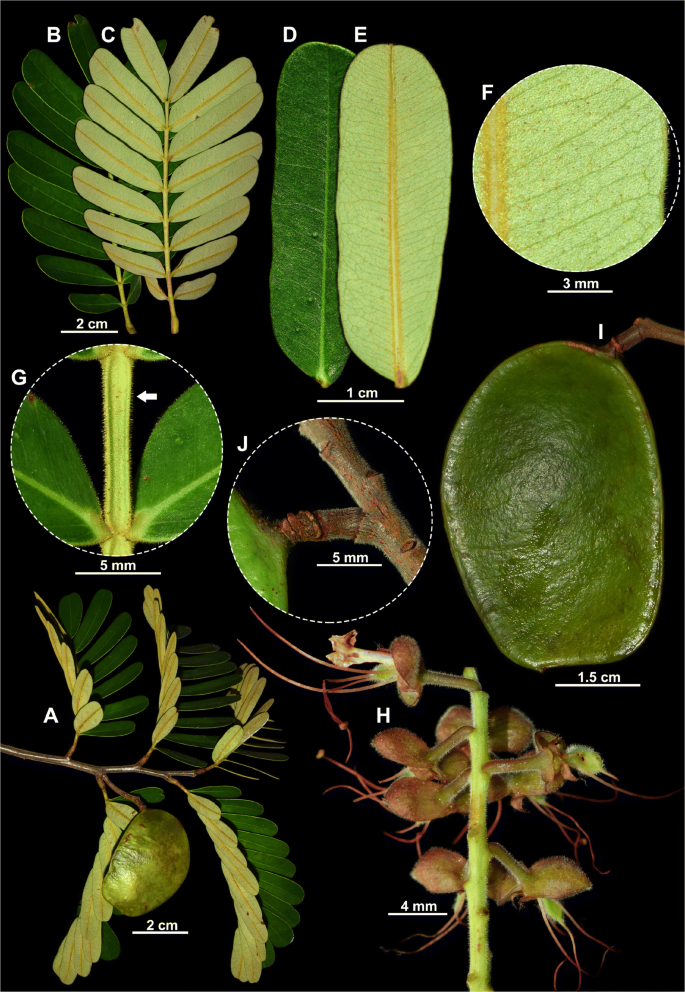This color photograph features a series of detailed images of various leaves and stems set against a black background. In the top left, two fan-shaped leaves are labeled B and C, one in dark green and the other in a lighter shade. Adjacent to these, labeled D and E, are two long, oblong leaves, also differentiated by their dark and light green hues. 

In the middle row, a closeup image labeled F focuses on the underside of a leaf, following which a photograph labeled G highlights a specific part of a stem with detailed inlets showcasing its intricate structure. Another closeup labeled J shows a twig with a branch, marked with a measurement of 5mm. This row also includes an image of a large green leaf, noted to be 1.5cm in size.

The bottom row features several more plants and parts: a multi-leaved branch labeled A, distinguished by a small green berry or fruit measuring 2cm, and a vertical plant, likely an orchid that hasn’t flowered, labeled H, with seeds or pods extending out, measuring 4mm. Each image provides intricate measurements and detailed inlets pointing to various anatomical parts, presenting a comprehensive study of plant material.